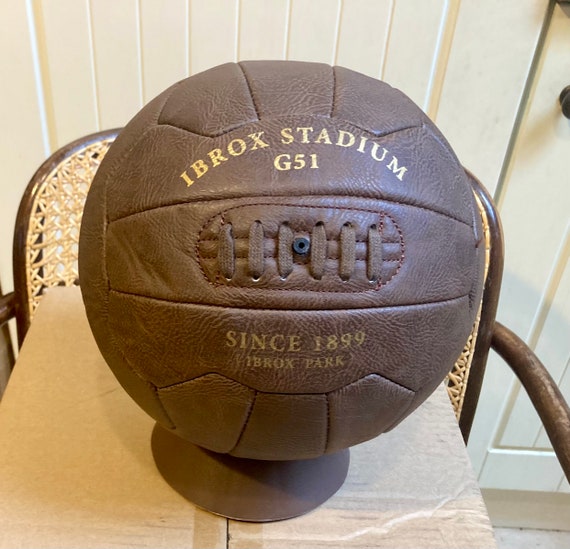The image depicts an antique, dark brown sports ball that resembles both a soccer ball and a football due to its round shape and prominent laces down the middle. The lettering on the ball, which appears worn and in a golden or brass hue, reads "Ibrox Stadium" in an arc at the top, "G51" horizontally below that, "Since 1899" under the laces, and "Ibrox Park" beneath that. The ball is well-preserved and displayed on a stand to keep it stationary. This stand is situated on a cardboard box, which, in turn, is placed on a chair. The background includes a knit chair and a white wall. The entire setup suggests the ball is a collectible, possibly an old version of a soccer or football, showcased carefully for display.